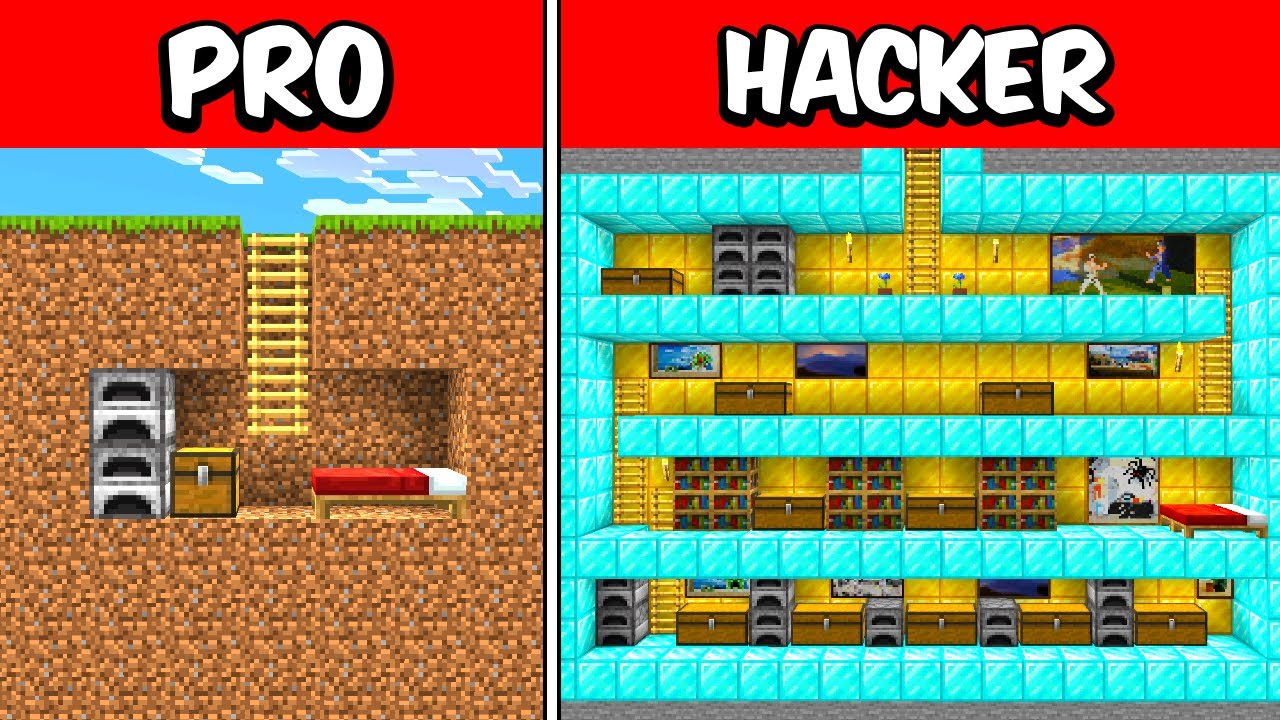**Left Image - Labeled "Pro":** The left panel showcases a pixel art game environment with a simple yet charming design. The scene features a grass-topped layer of dirt ground under a bright blue sky. A wooden ladder descends into a dug-out area, revealing a modest underground room. This room contains storage containers organized on the left side and a bed with a red blanket situated on the right. The top of this panel is marked with a red border and white lettering, prominently displaying the label "Pro."

**Right Image - Labeled "Hacker":** The right panel, denoted as "Hacker" in a similar red-bordered white text, presents a far more complex and elaborate underground world. This multi-layered design extends five to six layers deeper than the "Pro" version. The luxurious underground space is adorned with gold-colored walls illuminated by warm torchlight. The interior is richly decorated with paintings, bookcases, and features a sophisticated bluish tile for both flooring and walls, highlighting the contrast in complexity and opulence between the two images.